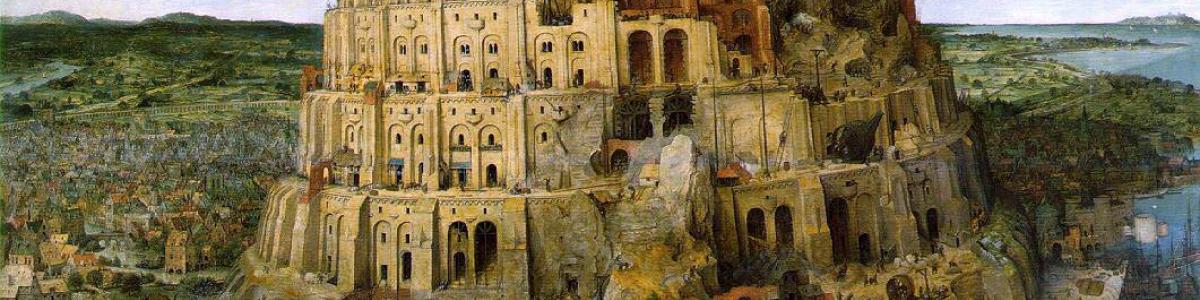This is an image, likely a classical painting, of the Tower of Babel, an ancient, monumental structure depicted in detailed, photorealistic style. The tower appears to be a massive, layered building carved from stone, extending upward with three distinct levels adorned with numerous windows and doorways. Despite its weathered appearance, the architecture is impressively well-preserved for its age, exhibited in a grayish-tan hue. The tower dominates the foreground, resembling a colossal castle-like edifice that forms the centerpiece of the composition. Surrounding the Tower of Babel, the painting captures a sprawling ancient cityscape with diverse buildings, including houses and huts, interspersed with verdant landscapes and blue waterways. The background reflects a mix of green and gray tones, with additional signs of civilization that highlight the monumental scale of the tower.